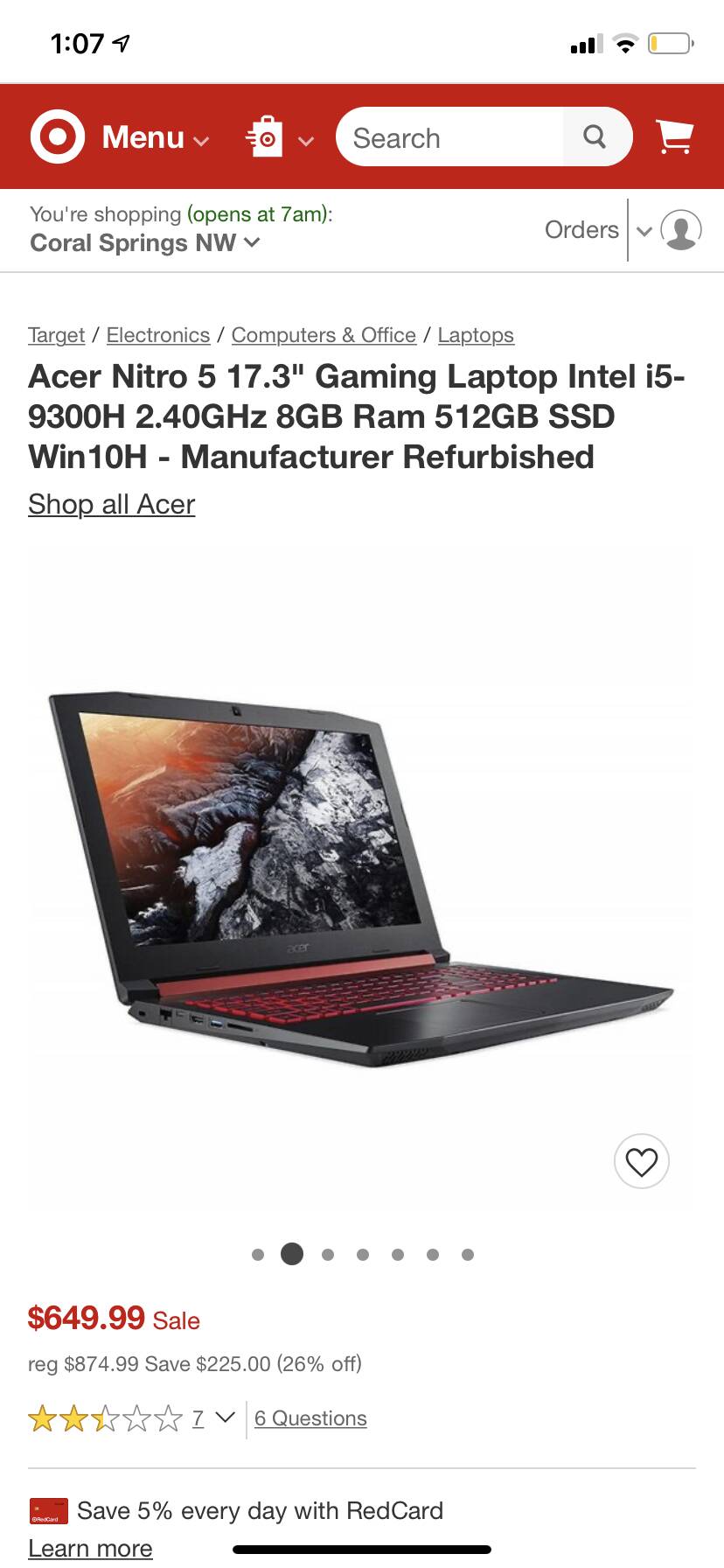A screenshot of the Target website taken on a cell phone. The time at the top of the screen reads 1:07, and the battery is almost depleted. The phone shows three bars of service and Wi-Fi coverage. The top of the screenshot features a red banner with the Target logo next to the word "Menu." Also displayed are icons for a shopping bag with the Target logo, a search bar, and a white shopping cart icon. Below, it indicates that the Coral Springs Northwest store opens at 7 a.m. There's an icon of a silhouetted person next to the word "Orders."

The webpage navigational path is detailed as "Target / Electronics / Computers & Office / Laptops." The main product featured is an "Acer Nitro 5, 17.3-inch Gaming Laptop" with specifications including Intel i5-9300H processor at 2.40 GHz, 8GB RAM, 512GB SSD, and Windows 10H. The laptop is manufacturer refurbished. There is a caption "Shop all Acer."

A photograph of the black laptop, which has a backlit keyboard with red lights, is shown. The screen displays an image of a volcanic landscape. The price is listed as $649.99 on sale, reduced from the regular price of $874.99, offering a savings of $225 or 26% off. The product has an average rating of two and a half stars from seven reviews, and there are six questions about the product. An additional prompt indicates that users can save 5% every day with a Target RedCard, with a link to learn more.